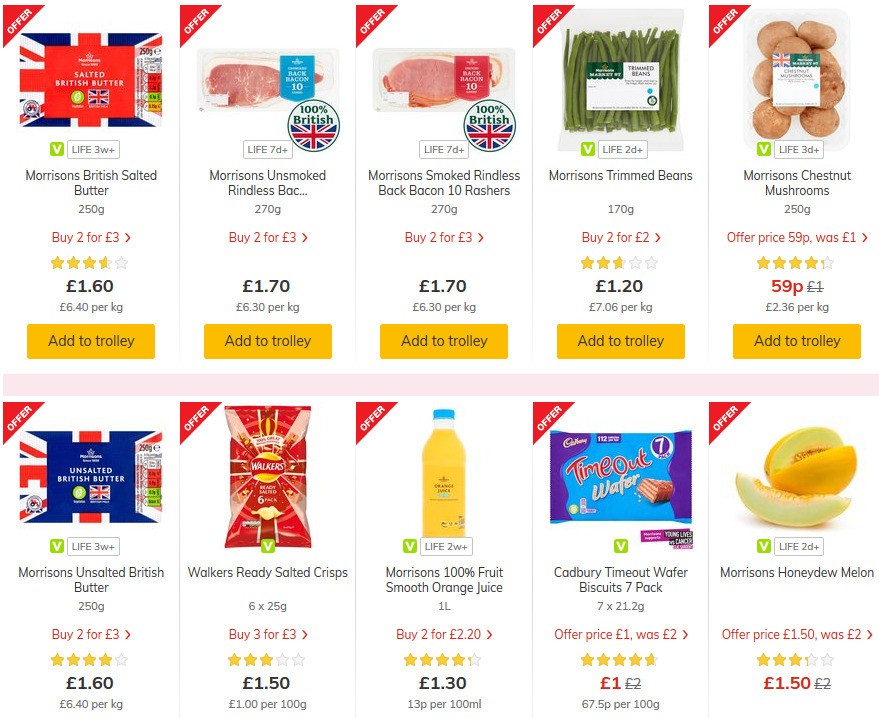This screenshot depicts a products page from a food retail website, showcasing a variety of food items arranged in a consistent format. Each item is displayed within its own box, organized in rows and columns, separated by thin vertical lines.

At the top left corner of each product box is a distinctive red triangle with the word "Offer" prominently displayed, indicating special deals. In the first row, each food item features an orange "Add to Trolley" button at the bottom for easy purchasing. 

The first product on the page is labeled as "Morrison British Salted Butter," weighing in at 250 grams. It comes with a special offer of "Buy 2 for £3" and is priced at £1.60 each. This item has received a rating of three and a half stars out of five.

Following this, the adjacent item to the right is "Morrison Unsmoked Rindless Bacon." This product's image is adorned with two tags: a blue one with the text "Back Bacon 10" and another featuring a British flag stating "100% British." It shares the same "Buy 2 for £3" offer and is priced at £1.70. The orange "Add to Trolley" button is also present at the bottom of this item.

The second row continues in a similar layout, although it lacks the orange "Add to Trolley" buttons at the bottom of each box. Each food product remains enclosed in its individual box with consistent spacing separated by vertical lines.